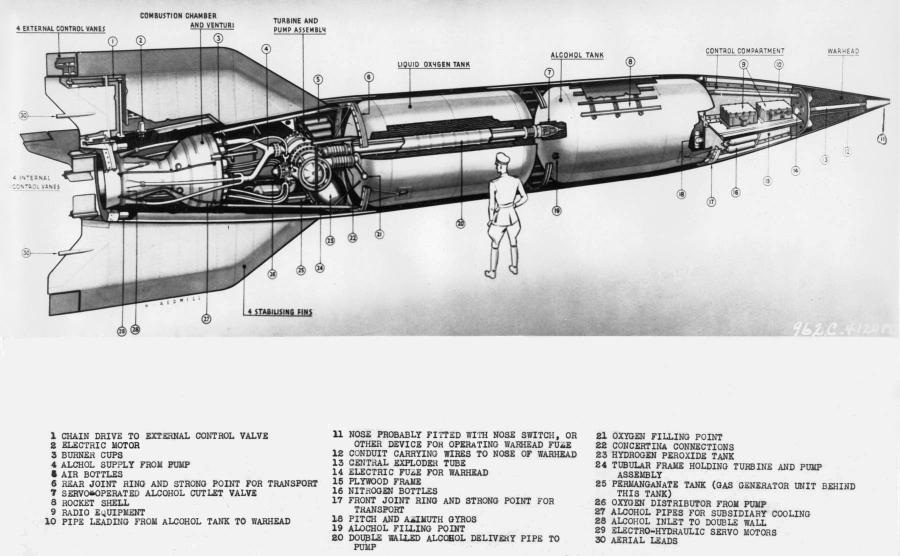This black-and-white schematic diagram depicts a large missile or rocket that appears to be an intricate design dating back to the 1930s or 1940s. Standing beside the missile is a man in a military uniform—wearing baggy pants, boots, and a hat—emphasizing the missile's immense size, which is estimated to be around 10 to 11 feet tall. The diagram features a detailed cutaway view, revealing the complex internals of the missile, including components such as the liquid oxygen tank, alcohol tank, electric motor, burner cups, and chain drive to the external control valve. There are numerous mechanical parts labeled numerically from 1 to 30, with corresponding names listed in a key below the image; for example, number 1 is labeled as "chain drive to external control valve," and number 30 as "aerial leads." The classic font and meticulous engineering details suggest that this diagram might be found in an old instructional manual or textbook.